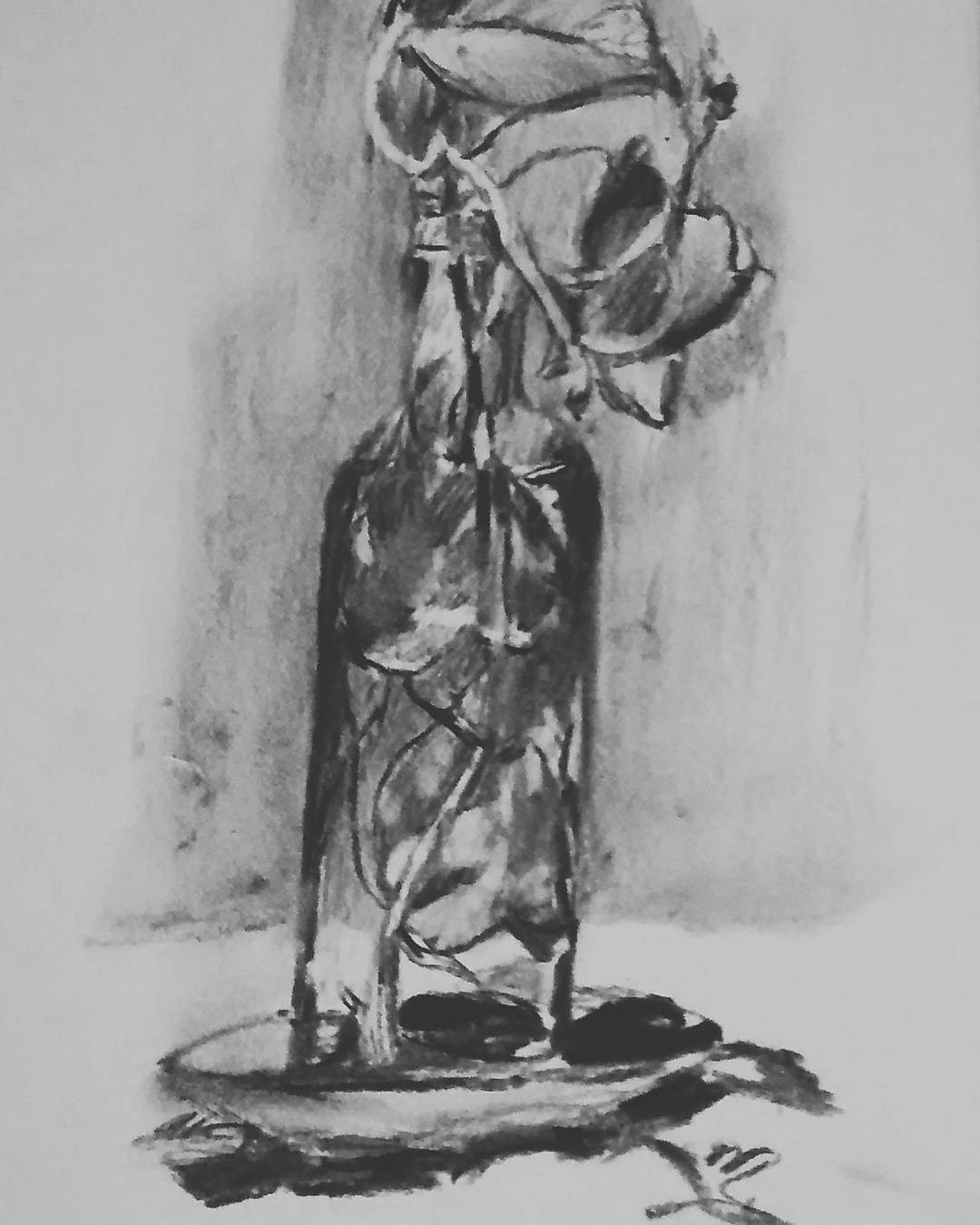The image captures an intricate piece of art centered on a white canvas, occupying the entire frame of the photograph. As the artwork extends beyond the visible boundaries of the image, it provides a sense of continuity and dimension. The focal point of the piece is a detailed depiction of a wine bottle, seemingly filled with flowers. The artwork is rendered entirely in black and white, presumably using charcoal to create varying shades and textures. Through the transparent glass of the wine bottle, one can observe the delicate flowers inside, while a separate stem, topped with a lily, extends gracefully out of the bottle's opening. Subtle shading in the background suggests the presence of shadows, adding depth to the composition. The wine bottle appears to be perched on a small plate that rests on a surface, grounding the scene in a realistic setting.